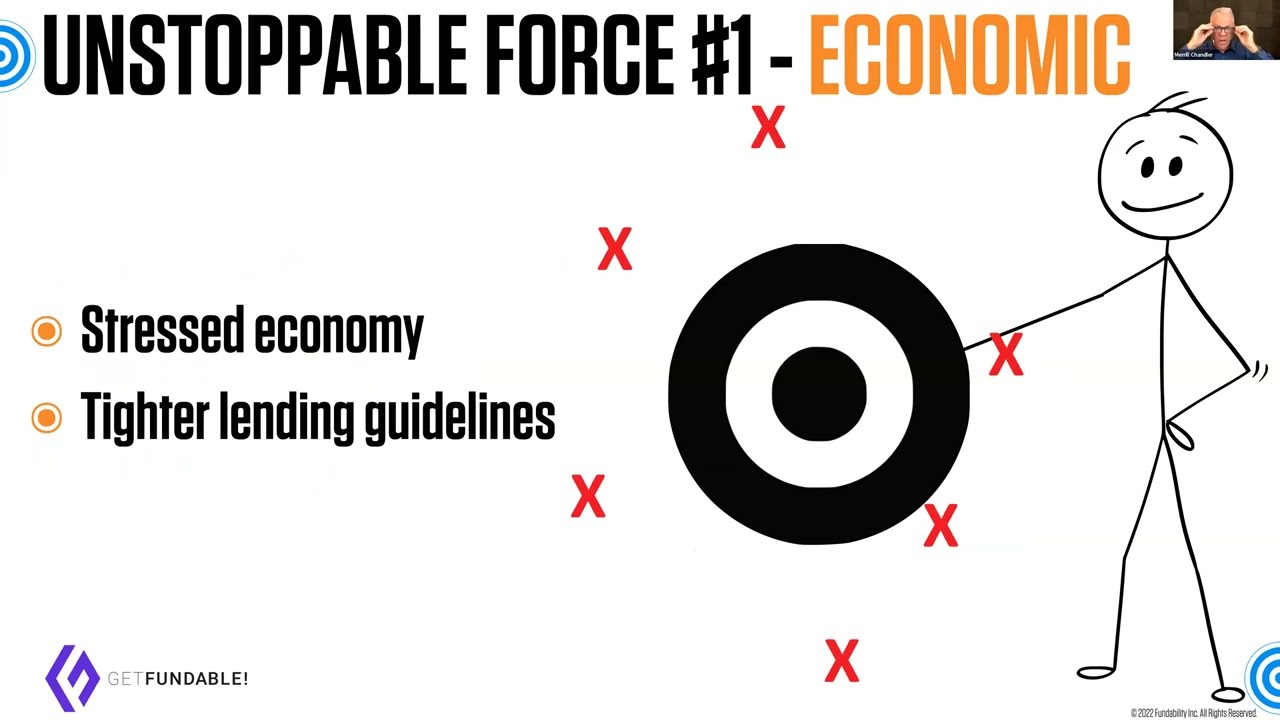This image is a detailed advertisement featuring various visual and textual elements. At the center is a prominent blue and white bullseye target with six red X's dispersed around it, symbolizing missed marks. Adjacent to the target is a black stick figure illustration, smiling and pointing at the bullseye. At the top, the headline reads "Unstoppable Force Number One" in black, followed by "– Economic" in orange text. On the left side of the image, two bullet points are listed: the first states "Stressed Economy" and the second "Tighter Lending Guidelines," both in orange. In the upper right corner, there is a small inset headshot of a man adjusting his glasses. At the bottom left of the image, a purple triangular logo displays the initials "GF" in white, beside the text "Get Fundable!" placed prominently. This ad combines photorealism and line art to emphasize economic challenges and promote lending solutions.